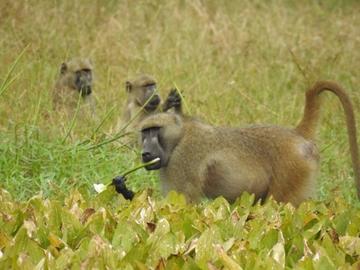This color photograph captures a peaceful scene in a grassy field populated by three tan baboons, identifiable by their black faces and hands. Prominently in the foreground is a side-profile view of one baboon, showcasing its raised tail and alert posture as it looks left. This baboon appears to be chewing on a branch. Behind it, two more baboons are partially obscured by the tall, greenish-yellow grass, visible only by their faces and hands. These two baboons seem to be examining and peeling something in their hands. The field is lush with large leaves scattered on the ground, enhancing the serene ambiance of the image.